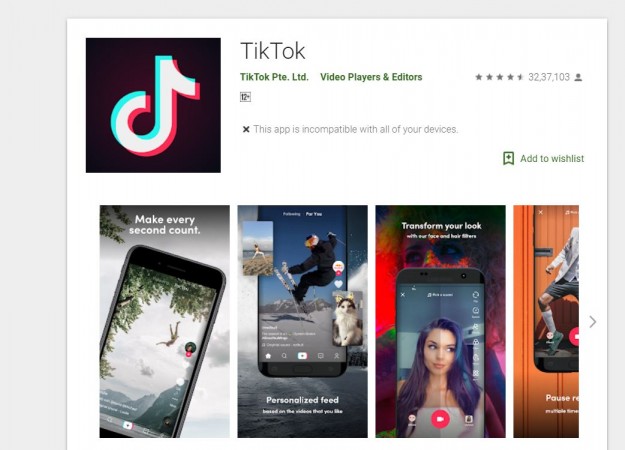The webpage displays a TikTok application overview on a white background. In the top left corner, the iconic TikTok logo is presented within a black square. Adjacent to the logo, the name "TikTok" is written in bold, followed by "TikTok PTE. LTD." in green text. Below that, "Video Players and Editors" is also highlighted in green.

An information section reveals the app’s rating and user base, depicting stars and a membership count of 32,103. A box indicates that the application is recommended for users aged 12 and up. However, an "X" signifies that the app is incompatible with the viewer's devices. There’s also an option labeled "Add to Wishlist."

At the bottom, four equally divided rectangles display a series of promotional images. The first image shows a person free falling into water, accompanied by the caption "Make Every Second Count." The second rectangle features a skier, with the label "Personalized Feed," and includes small inserts of a cat and a person practicing yoga on a beach. The third image showcases a girl with the caption "Transform Your Look." The fourth rectangle is partially obscured, making its contents unclear.